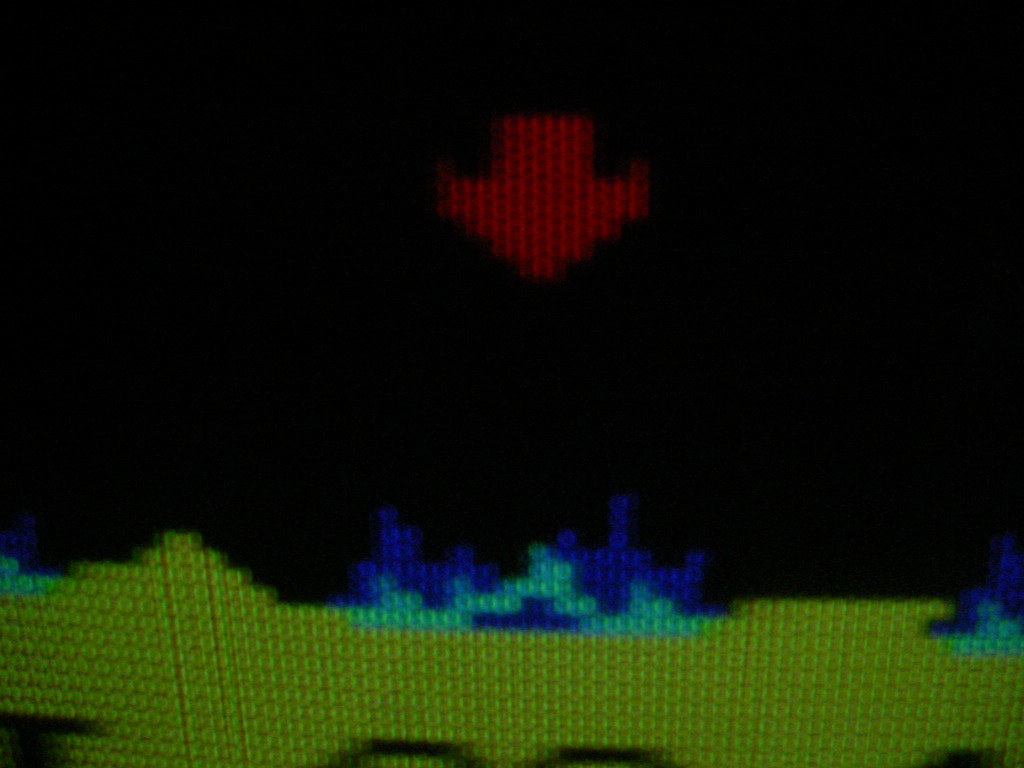The photograph resembles a screenshot from a vintage video game, characterized by its distinctly pixelated graphics. The image is horizontally oriented and predominantly filled with solid black. At the bottom, a horizontal stretch of light green terrain spans the width of the frame. The terrain appears relatively even, with a few minor undulations. Scattered across this green ground are several dark blue plants featuring lighter turquoise patches, adding to the pixelated aesthetic. Centered above this terrain, a conspicuously pixelated red arrow points downward, specifically targeting one of the bushes. The arrow's vibrant red contrasts sharply with the darker hues of the surrounding elements, drawing immediate attention to the indicated spot.